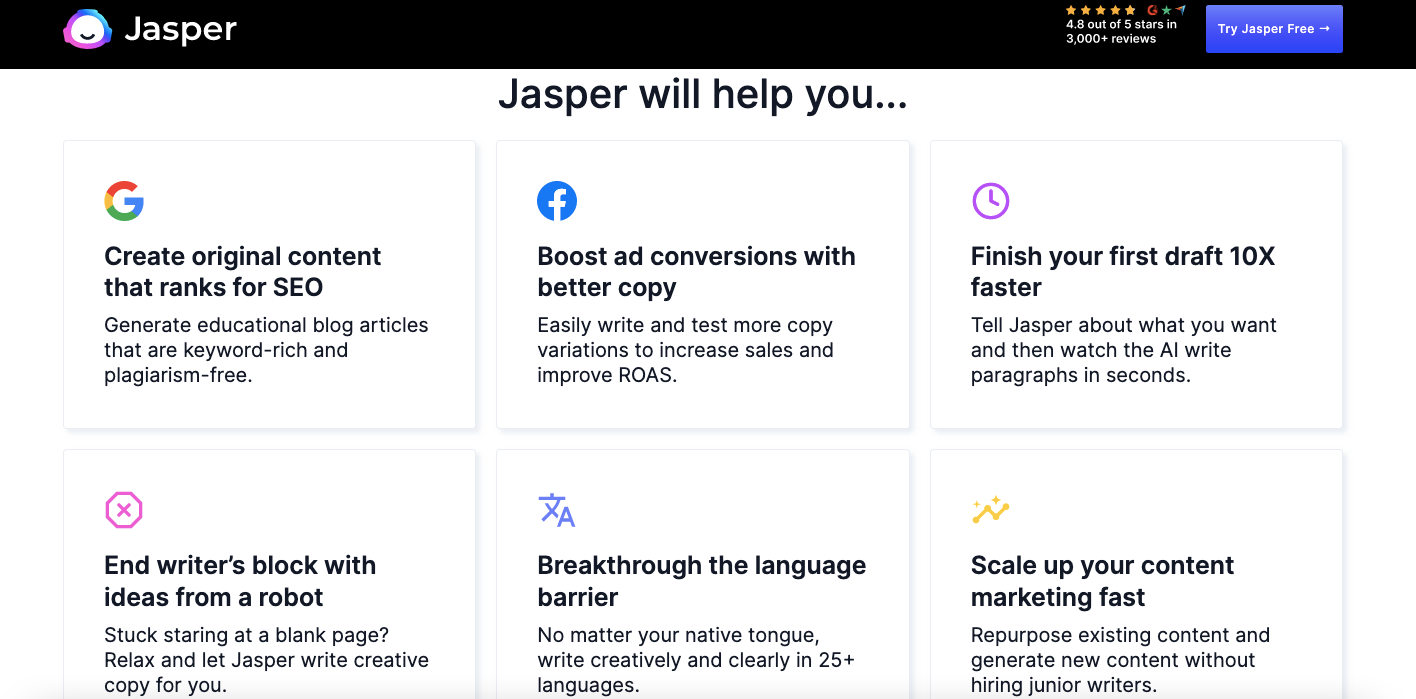This is a screenshot from the Jasper website (or possibly its application). The upper left of the screen features the Jasper logo, positioned on a black bar that spans the width of the page. The logo is distinctive, featuring a smiley face within an oval-white inner section, encircled by an outer ring with a gradient from pink to blue transitioning from the lower left to the upper right.

In the upper right corner, there is a rating displayed: 4.8 out of 5 stars from 3,000 reviews, accompanied by a button labeled "Try Jasper for free."

Beneath the black bar, in the white section, there is a headline that reads "Jasper will help you...". Six options are displayed below this headline in a grid format, with three options across and two down.

1. The first option features the Google logo and reads: "Create original content that ranks for SEO. Generate educational blog articles that are keyword-rich and plagiarism-free."
2. The second option, marked by the Facebook logo, states: "Boost ad conversions with better copy."
3. The third option displays a purple clock icon with the text: "Finish your first draft ten times faster."
4. Directly below, there is an "X" button with the caption: "End writer's block with ideas from a robot."
5. Another option labeled "Translation" reads: "Break through the language barrier."
6. The final option, illustrated with a graph icon, promises: "Scale up your content marketing fast."

This screenshot illustrates that Jasper is an AI solution designed to assist users in creating superior copy, enhancing productivity, and improving marketing outcomes.